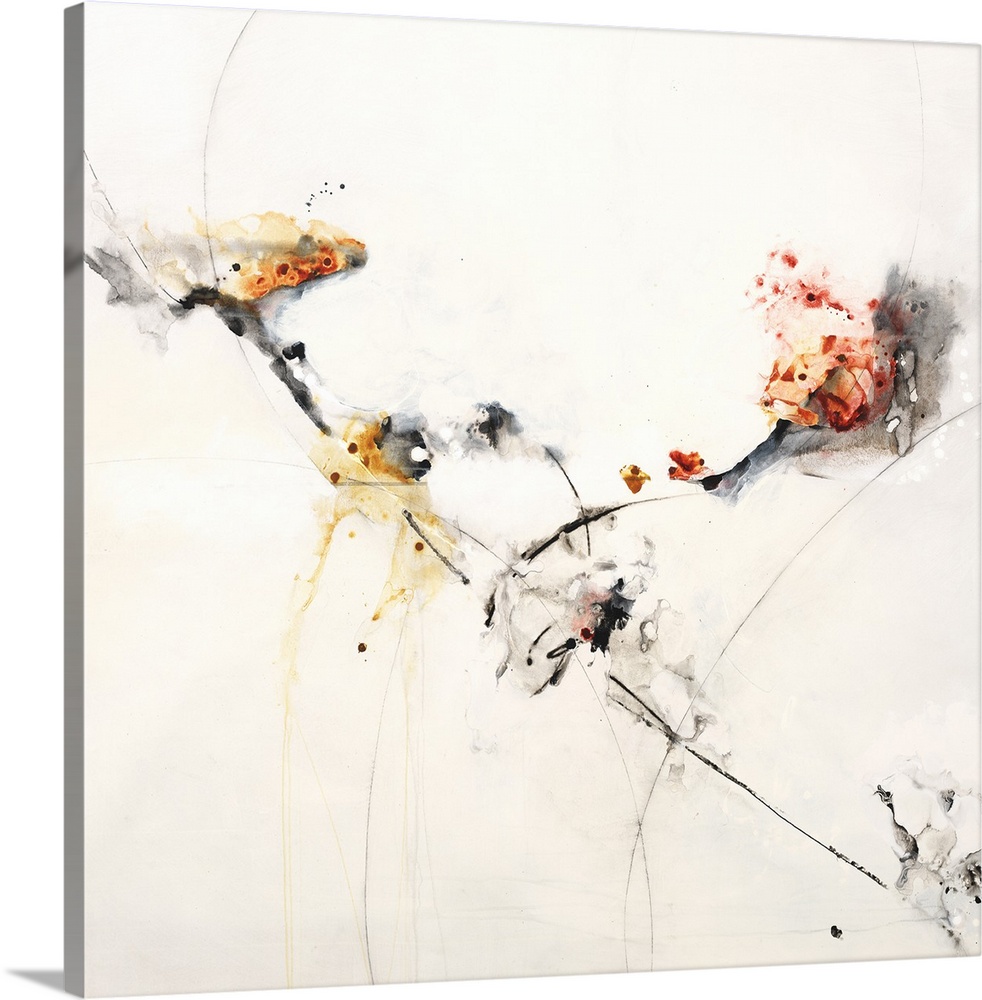This image is a stock photo of an abstract painting on a perfectly square, stretched canvas. The background is primarily white, though not perfectly so, with subtle smears of color and a light marbling effect in gray. The painting features abstract splatterings and smeared areas in the center that introduce various colors and textures, primarily using shades of black, yellow, orange, and red. The central design, open to subjective interpretation, somewhat resembles a flower. The paint has been splattered and there is noticeable texture where the paint is raised. Thin black lines and tan lines traverse the canvas, running diagonally from the top left corner to the bottom right corner, and branching off to the top right. Additionally, a distinctive white and red ball, outlined in black, is located at the top right, while a black and brown section with some red appears at the top left and center, forming a Y-shape. Another black splatter can be seen in the bottom right corner, enhancing the dynamic, abstract nature of the artwork.